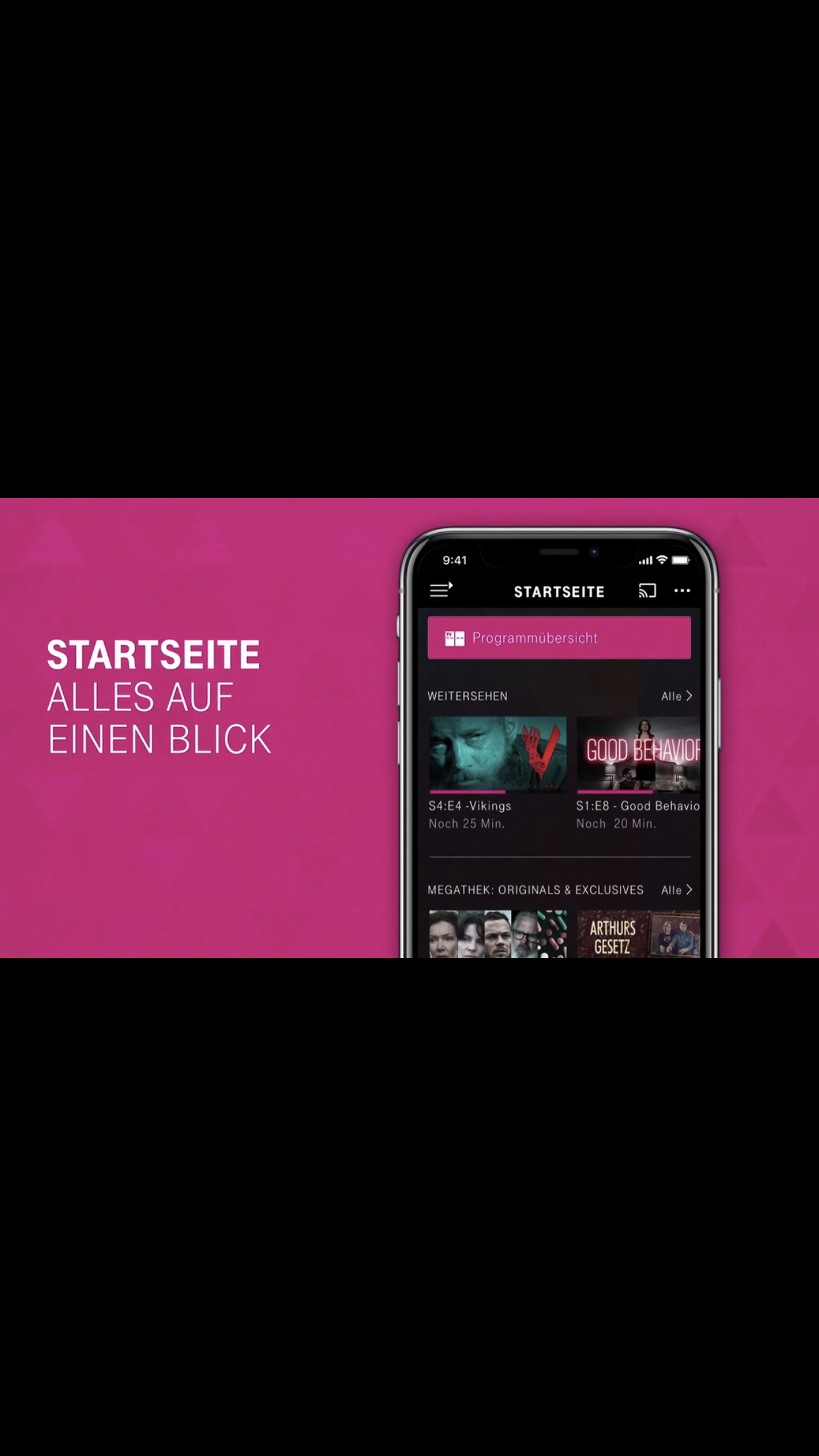The image is an advertisement for a mobile app, set against a predominantly black background. In the center of this dark backdrop, a hot pink rectangle houses a smartphone, likely an Apple iPhone 8 or 9. The phone's screen displays a user browsing through TV shows, with "Vikings" (Season 4, Episode 4, 25 minutes) and "Good Behavior" (Season 1, Episode 8, 20 minutes) prominently featured. Below the shows, the text reads "Meek Ethic, Originals and Exclusives." Additionally, there are images of people's faces. To the left of the phone, captions in German include "Start Site" and "Alice Auf Einen Blick." The colors in the ad are black, pink, white, green, blue, and brown, contributing to the visual appeal. Overall, the advertisement is likely for a streaming app, with the imagery and text suggesting it could be similar to HBO Max or Hulu.